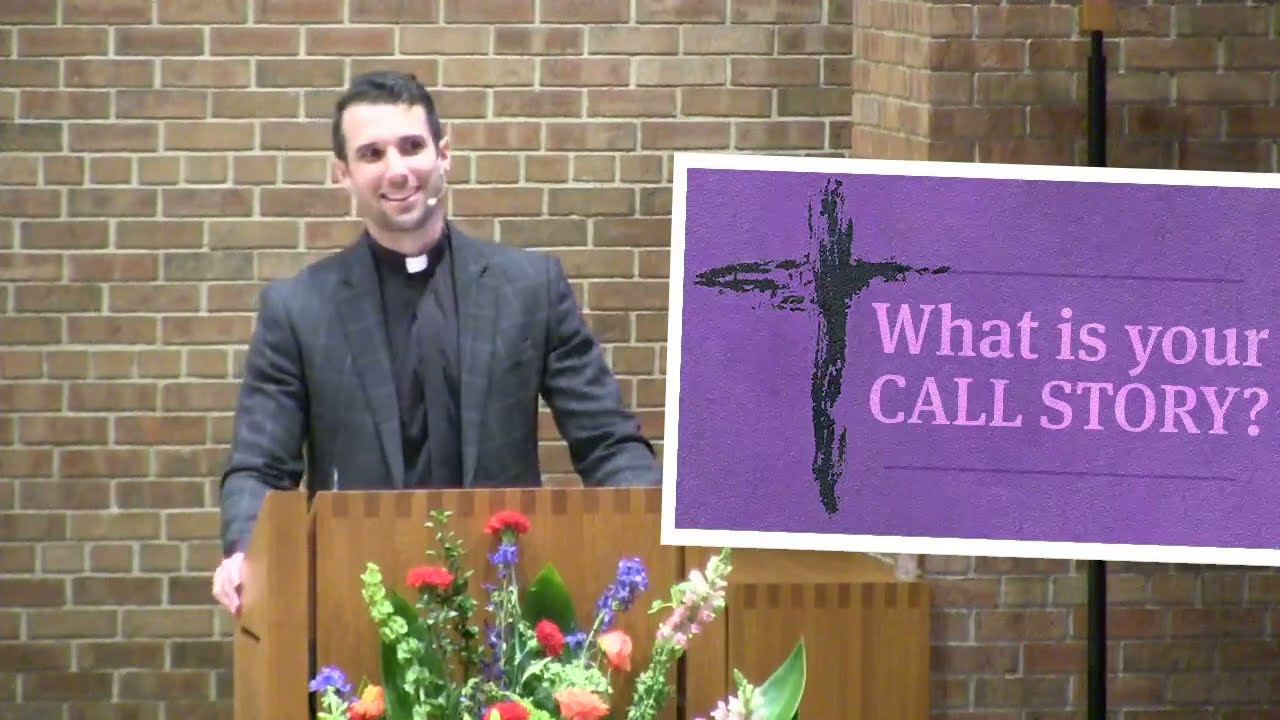In this color image, a light-skinned priest stands behind a wooden podium, which features a vibrant floral arrangement consisting of red, pink, purple, and various other colored flowers. He has short dark hair and is smiling warmly as he looks slightly to the right of the image. The priest is dressed in a black clerical shirt with a white collar and a dark sport jacket with a subtle square pattern. He wears a headset microphone that projects in front of his mouth and grips the side of the wooden podium with his right hand.

The background is a brown brick wall that adds texture to the setting. On the right side of the image, a purple rectangular sign with a white border is prominently displayed. The sign features a black abstract painted cross and two lines of lighter purple text that read, "WHAT IS YOUR CALL STORY?"